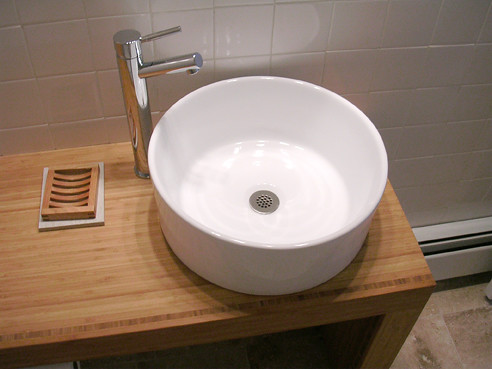A pristine white, standalone sink sits elegantly on a light brown wooden cabinet. The sink features a circular, silver drain with multiple small holes at its center. Rising from the upper left side of the sink is a sleek, silver faucet, which extends outward to hover just above the basin. The faucet is distinguished by a small rod on its top, protruding to the right. Positioned close to the cabinet's right edge, the sink is nestled in the corner of the space. The backdrop showcases a wall adorned with gray ceramic tiles, reflecting a soft light from the sink, creating a bright spot on the surface. Beneath the cabinet, a shadowy square recess is visible, hinting at storage space within. To the left of the sink rests a rectangular wooden object, featuring sloping bars across its center, made from matching wood. This wooden piece is placed atop a light gray fabric, which is slightly larger than the wooden object itself, adding a touch of texture and contrast to the setup.